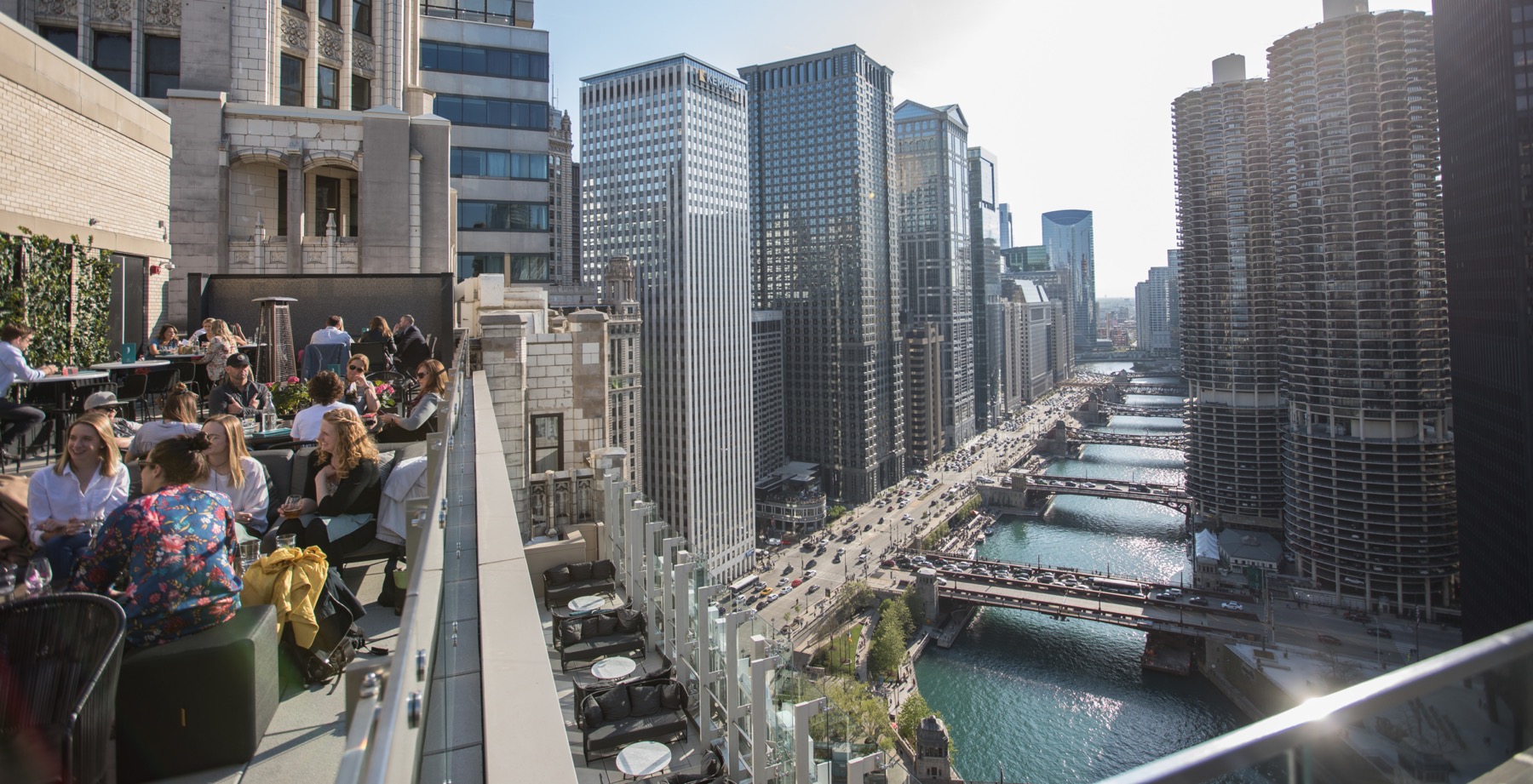The image depicts a sprawling cityscape, likely Chicago, from an elevated perspective with a bustling outdoor dining area in the foreground. On the left side of the image, a large balcony or patio is crowded with people sitting at numerous tables and chairs, likely part of a bar or restaurant. Just below this balcony, there are more tables and chairs on a lower level, suggesting an expansive multi-tiered dining facility. The cityscape features many high-rise buildings, including twin towers on the right, creating a dramatic skyline. The central focus is a wide river or bay with multiple bridges and a large highway running parallel to it, carrying heavy traffic and connecting various parts of the city. The highway appears to be a substantial six-lane road with numerous cars. Additionally, vertical and horizontal roads intersect the scene, leading towards the river and beyond. The background includes a mix of trees and urban landscapes under a sky that is partly cloudy, with patches of blue peeking through, indicating a bright and sunny day.